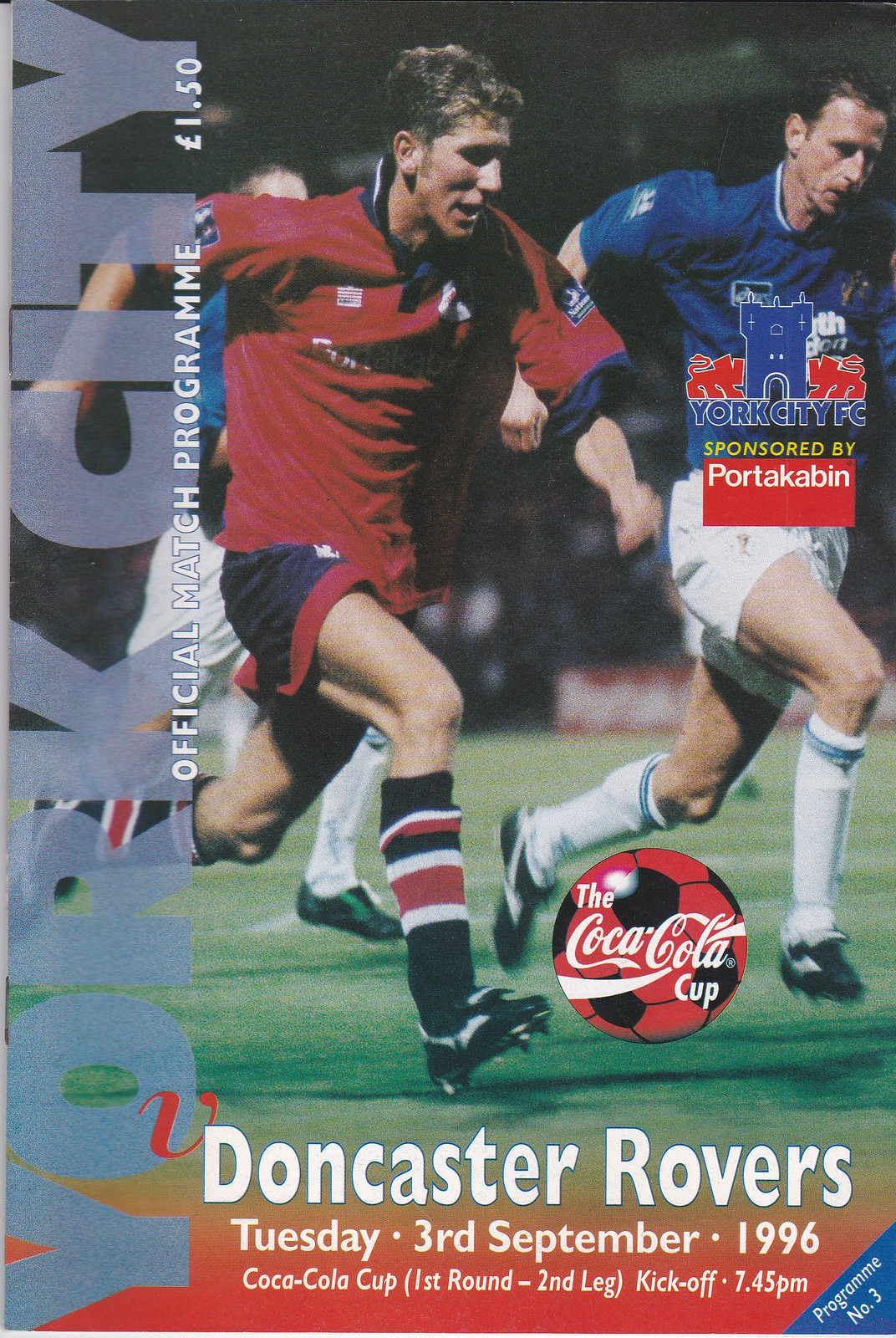The image is a detailed advertisement for a soccer event, featuring two players in mid-action. The focal point is a player in a red jersey and black shorts, accented with red, black, and white shin guards and socks, kicking a red and black soccer ball with the Coca-Cola Cup logo on it. Opposed to him is a player in a blue jersey, white shorts, white socks over his shin guards, and black cleats. The ball, prominently displayed, appears slightly glossy and possibly edited into the image. The advertisement includes text details: "Doncaster Rovers, Tuesday, September 3, 1996," "Coca-Cola Cup, First Round, Second Leg, Kickoff 7:45 p.m." Additionally, it mentions "York City Official Match Program $1.50" and "Program No. 3" in a blue triangle at the bottom right.